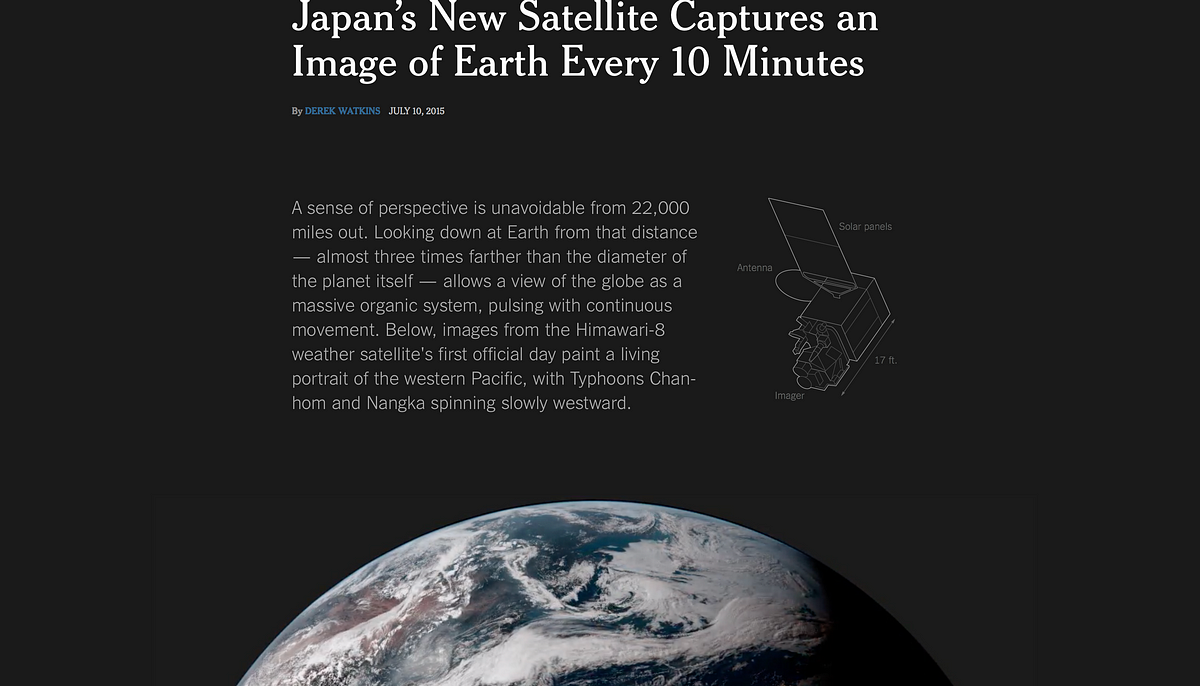A detailed caption for the described image could be:

---

**Caption:**

A screenshot showcases a detailed article on Japan's innovative weather satellite, Himawari-8, featuring white text on a stark black background. Authored by Derek Watkins and dated July 10, 2016, the article delves into the satellite’s groundbreaking capability of capturing an image of Earth every 10 minutes from an astonishing distance of 22,000 miles – nearly three times the planet's diameter. This striking perspective offers an unparalleled view of the globe, portraying it as a dynamic, interconnected system teeming with continuous movement. 

Specifically highlighted are images from Himawari-8’s first official day, vividly capturing the Western Pacific teeming with two powerful typhoons, Chan Hom and Nangka, spiraling slowly westward. This depiction underscores the satellite’s primary focus on weather observation.

Adding to the textual narrative, a small white illustration of the Himawari-8 satellite is positioned to the right of the text. The diagram meticulously labels key components such as the solar panels, antenna, and imager, emphasizing the unit's dimensions with length arrows. 

The bottom of the screenshot features an evocative image of Earth set against a dark void, reinforcing the sense of scale and the continuous, fluid nature of our planet's atmosphere as captured by this advanced satellite.